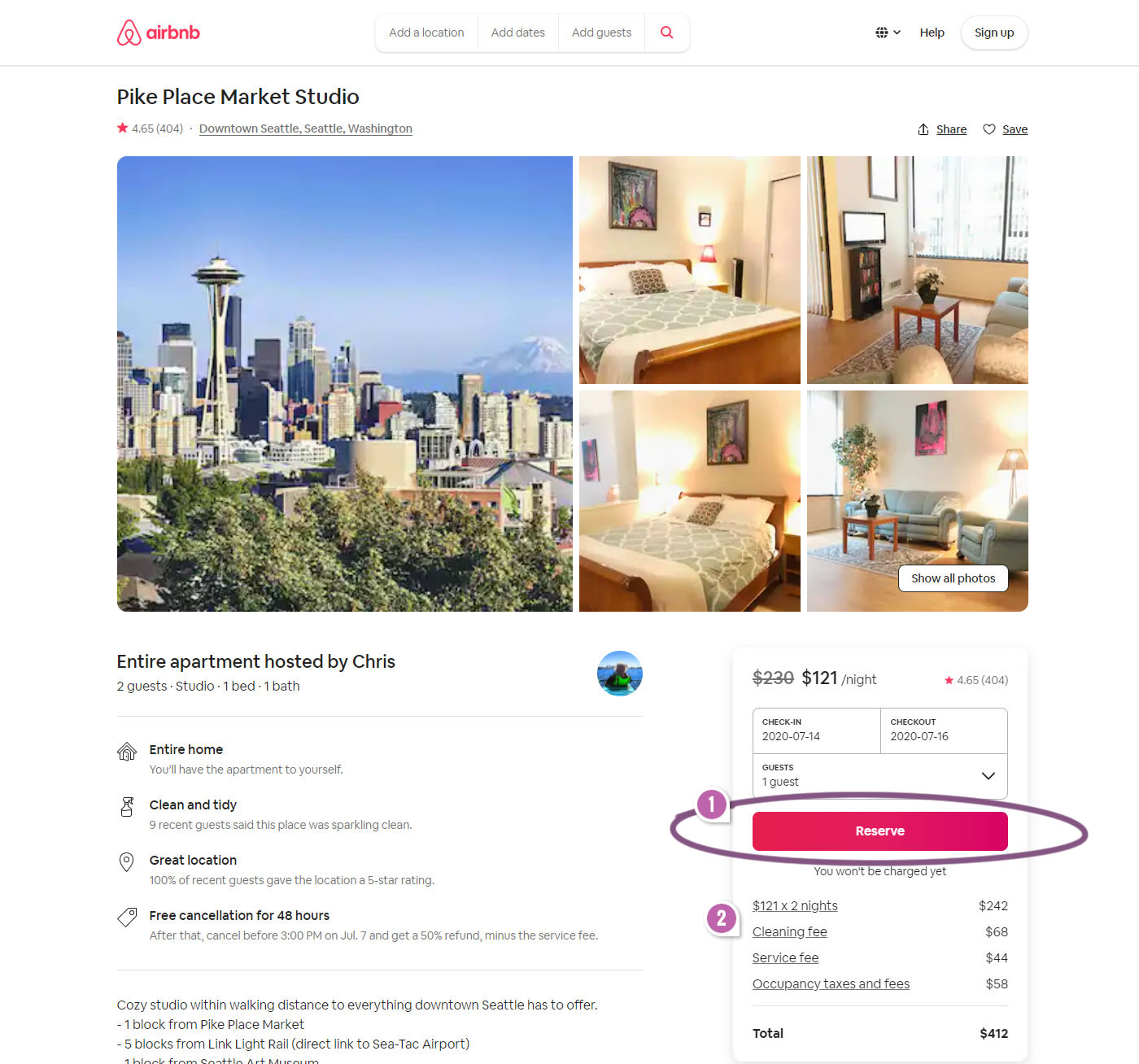Screenshot of Airbnb listing for a Pike Place Market studio in downtown Seattle, Washington:

The left side of the screenshot prominently features a large image capturing a stunning overview of Seattle, extending out to the surrounding mountains. The right side showcases four smaller images providing a detailed glimpse into the cozy studio apartment.

1. The first image reveals a beautifully decorated bedroom with a walnut bed, dressed in soft grey covers. A vibrant, multicolored painting adorns the cream-colored wall behind the bed, adding a splash of color to the elegant setting.
2. The second image highlights a quaint table set on a stylish rug, positioned beside a small bookcase. Large windows bathe the room in natural light, with a beige armchair's arm peeking into view.
3. The third image offers another angle of the bedroom, displaying its comfort and inviting atmosphere from a different perspective.
4. The fourth image presents a cozy living area featuring two grey couches, a lovely table with a floral display and a lamp, exuding a warm and welcoming vibe.

Additional details about the listing:
- Hosted by Chris
- Accommodates 2 guests, with 1 bed and 1 bath
- You have the entire apartment to yourself
- Clean and tidy space
- Excellent location with proximity to Pike Place Market
- Free cancellation within 48 hours
- The rate is $121 per night

In the screenshot, someone has begun the booking process, indicated by a circled reservation button showing the number "1" on a purple dot. Below it, the breakdown of costs includes $242 for two nights, alongside a cleaning fee, a service fee, and occupancy taxes and fees.